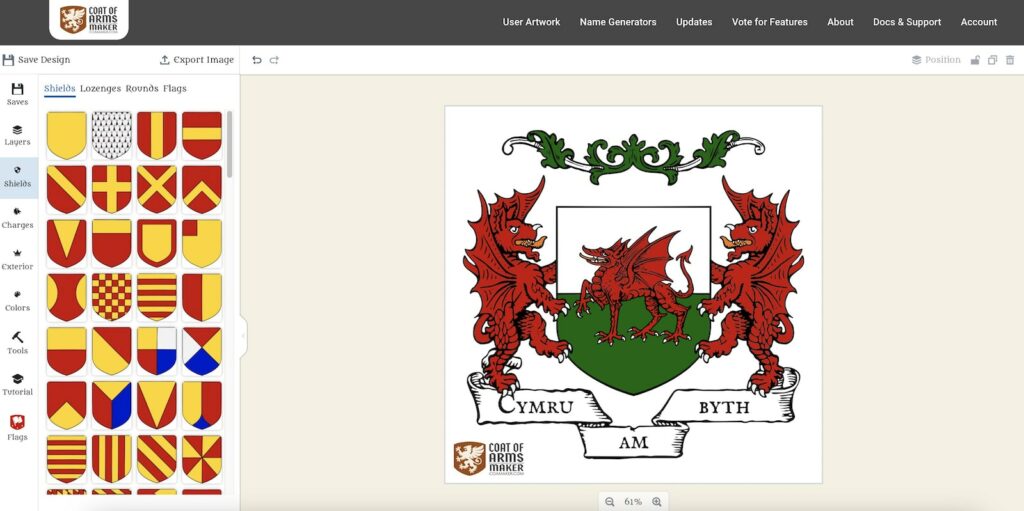The image is a detailed color screenshot of a website featuring a program for designing a family crest or coat of arms, titled "Coat of Arms Maker." The primary focus is a large white and green heraldic shield at the center, adorned with a prancing red dragon facing left. Flanking the shield are two additional red dragons. Above the design, the banner reads "Cymru Am Byth," a phrase that appears to be in Welsh. The image includes a top black navigation bar with various options such as User Artwork, Name Generators, Updates, Vote for Features, About, Docs and Support, and Account. Additionally, there are icons for exporting images and saving designs. To the left of the main image, there is a column displaying several rows of different heraldic shields in various colors, predominantly red and yellow, with some black, white, and blue elements.